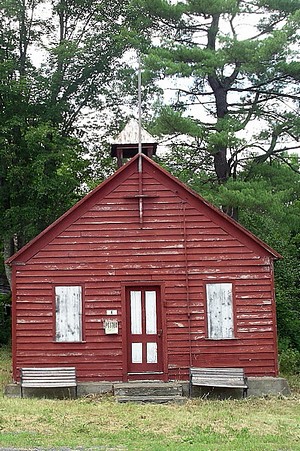The image captures a small, aged structure which appears to be either a cabin, house, or possibly even a schoolhouse or business. The building is primarily red, albeit with significant discoloration showing patches of white where the paint has weathered away. It features a V-shaped roof topped with a gray metal pole, potentially for hanging a sign, suggesting it could have functioned as a business at some point. 

The front door, adorned with rectangular patterns painted white, is flanked by two windows also trimmed in white. Below each window, there's an old wooden bench showing signs of neglect and possibly unsafe for sitting. Two steps lead up to this front door. Surrounding the building is wild, somewhat overgrown grass, with a few longer patches giving it a rugged appearance. The backdrop includes a cloudy sky and numerous trees full of leaves, enhancing the rustic and somewhat abandoned feel of the scene.